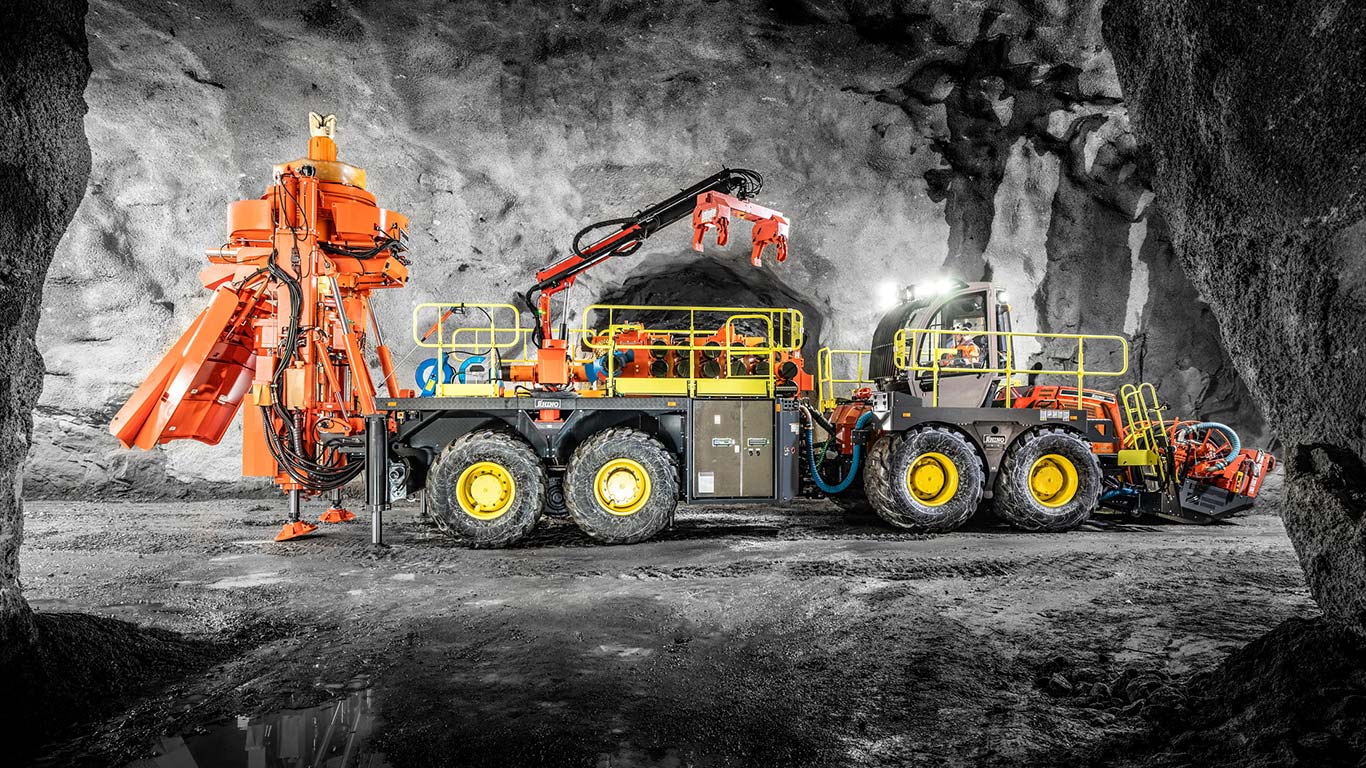The image depicts a large, intricate construction machine situated in what appears to be a dimly lit cave or mine, evidenced by the stone and rock walls on all sides and a rocky ground. The machine, predominantly black and yellow, is composed of multiple connected segments and has a rugged, industrial look. The primary vehicle is equipped with four large tires with deep treads and features a yellow, railing-like structure on top, providing a safety barrier. The cab where the operator sits is illuminated by bright lights, and the vehicle itself is oriented towards the right side of the image.

Attached to the main body of the vehicle is an additional section that houses more machinery. Among these is a prominent orange and black claw-like device, raised at an angle, designed for grabbing or lifting materials; it has two distinctive grabber claws. Another notable feature is the red apparatus at the front, which descends downward, possibly for drilling or stabilizing purposes. Both parts of the machine are connected, with visible hoses and ladders adding to the complex design.

In the background, there is a tall orange structure with two legs and sliding mechanisms extending from it, further indicating a sophisticated setup aimed at heavy-duty operations within this subterranean environment. The overall scene suggests a bustling, high-intensity construction or mining activity deep underground.